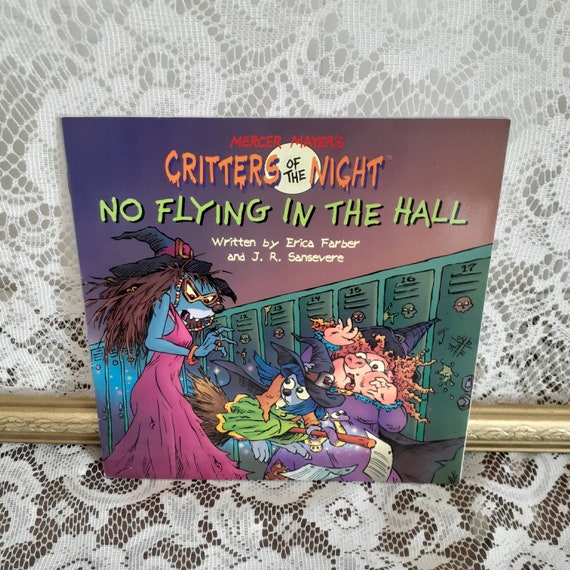The image features a children's book titled "Mercer Mayer's Critters of the Night: No Flying in the Hall," written by Erica Farber and J.R. Sansevier. The book is set against a white lace tablecloth, possibly a tablecloth draped over a table, with a visible edge of a gold frame or molding strip along the bottom. The book cover displays a vibrant illustration: on the left is a witch-like figure with blue skin, glasses, and creepy brown hair, dressed in a pink dress and a black witch hat. This character appears to be a possum. Also depicted is a dog-like creature flying on a broomstick, wearing a witch hat and cape, and a pig in a purple dress cowering in fear. The background showcases green school lockers, adding to the scene's spooky school setting. The top of the cover features the title "Mercer Mayer's Critters of the Night" in bold letters, with "No Flying in the Hall" written below in green text. The authors' names are listed in white text underneath. The background gradient transitions from purple on the left to a dull purplish-brown on the right.